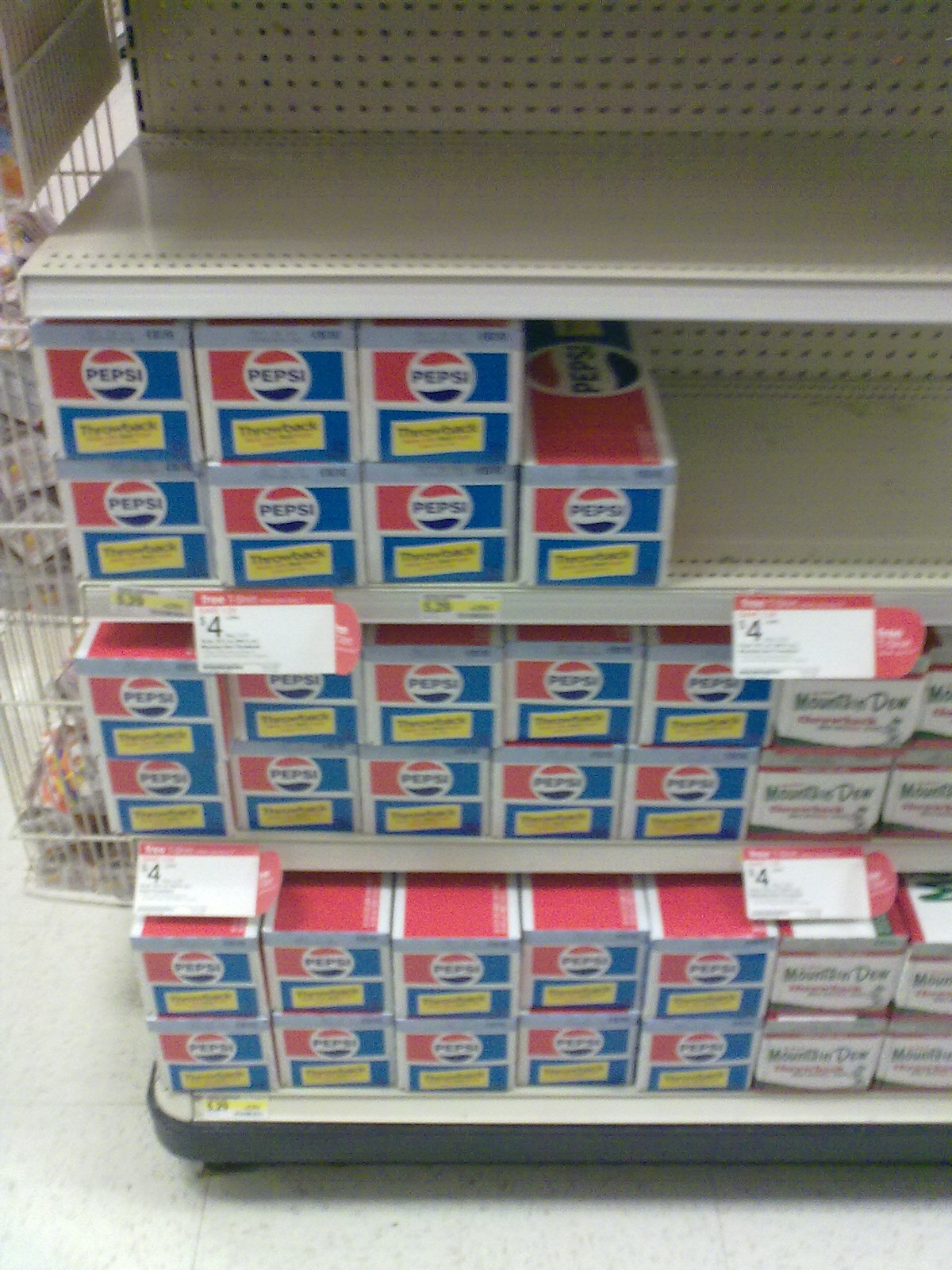The image depicts a supermarket aisle stocked with various beverages. Prominently displayed are numerous cartons of Pepsi, organized across several shelves. Analyzing the shelves, the top shelf is empty, the middle shelf is half-empty, while both the second to last and bottom shelves are fully stocked. Each box, potentially containing 12 cans of Pepsi, is priced at $4, which appears to be an affordable rate. Adjacent to the Pepsi cartons, there are also boxes of Mountain Dew, though the image is slightly blurry, making the branding less distinct.